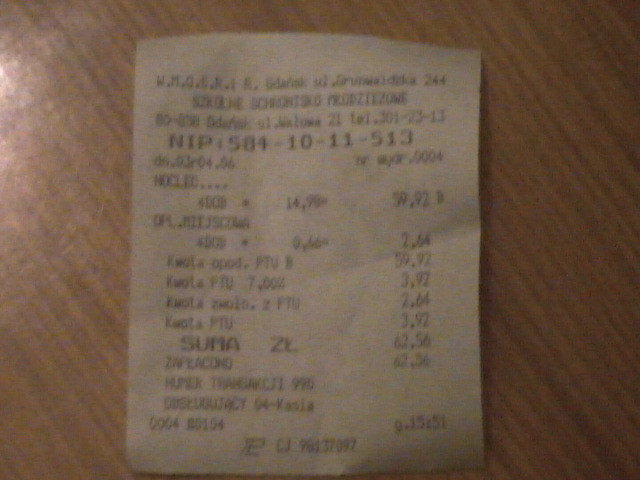This image depicts a small, somewhat worn-looking receipt with extensive text printed on it. The receipt, though partially legible, prominently features the letters "WMO" at the top, followed by a sequence of numbers. It appears to be itemized, with several entries listed beneath the header. Notably, many of the item names seem to begin with the letter "K," which might suggest a recurring product or a specific category. The right-hand side of the receipt displays various prices, culminating in what seems to be a total amount at the bottom. The receipt is placed on a simple, brown wooden table, which, although not particularly expensive, adds a rustic touch to the scene.